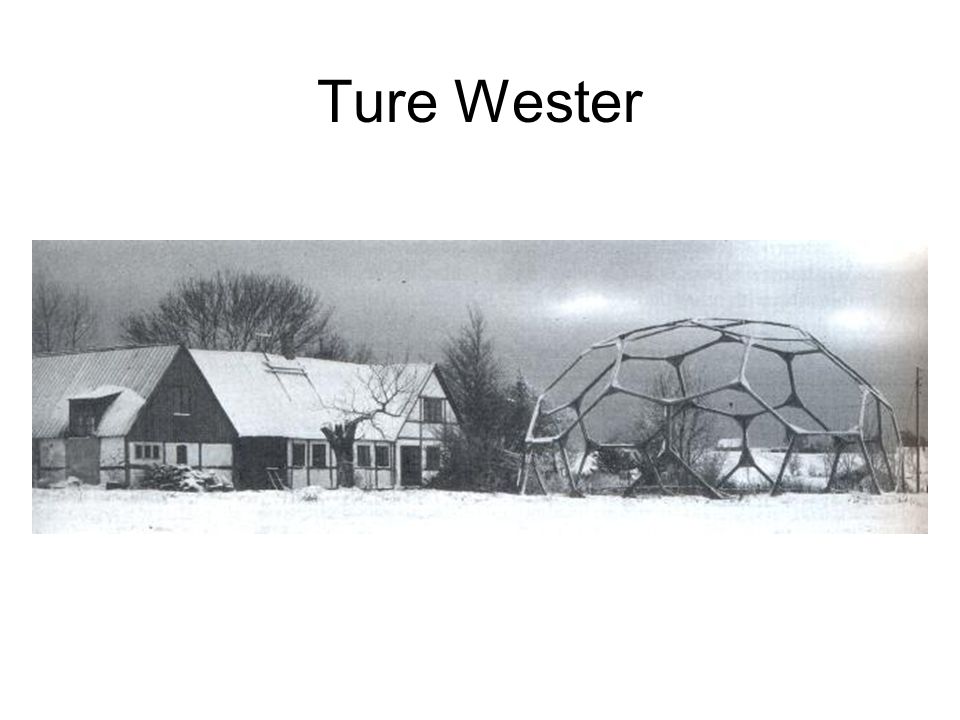In this narrow, horizontal, black-and-white winter scene, a large building with a snow-covered gabled roof stands prominently on the left. The building could be an inn or a school, evoking a sense of community with its welcoming structure. To the right, a geodesic dome jungle gym—resembling open sets of hexagons hooked together—sits in a snowy open area, hinting at a playground atmosphere. The overcast sky suggests more snow is imminent, and the ground is already blanketed in white. Deciduous trees with bare branches surround the scene, adding to the wintry bleakness. In the background, on the right, there appears to be a lake or a snow-covered hole. Above the image, the text "Ture Wester" is printed in black on a white background, with a big 'T' and 'W', indicative of the photographer or the image’s title.